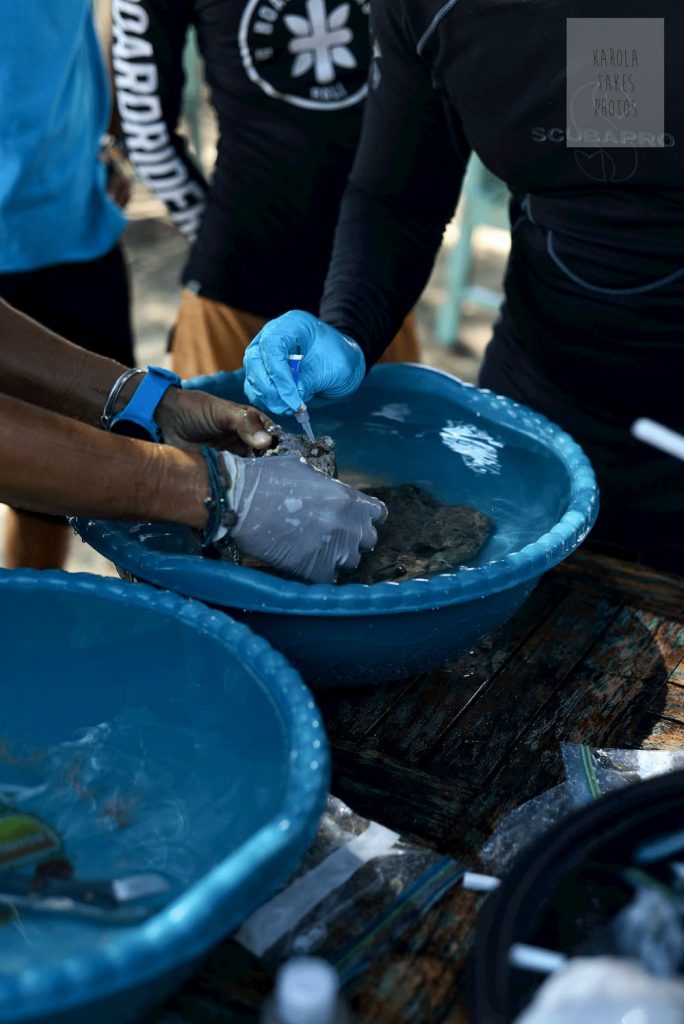In the photograph, several individuals are gathered around portable basins, outfitted in what seems to be a mix of biking and scuba gear. Starting from the back top left, there is a man wearing a blue shirt and black shorts. The visible portion of him spans from just below his neck to above his knee, with his leg in clear view. Next to him stands another individual, identifiable by the logo on their black shirt, featuring a white circle and a leaf. The long-sleeve shirt's sleeve has partially visible lettering, possibly reading "Board Rider" although some letters are cropped out.

In the foreground, a person dressed in scuba gear has their back turned slightly to the camera, the word “Scuba Pro” clearly displayed on the outfit. They are wearing blue latex gloves and are pictured squeezing something from a container into the water of a basin that contains a rock.

To the right, another individual's hands, also gloved, are submerged in the same basin, methodically working. Additionally, there is a second basin to the left, filled with water and an indistinct object at the bottom. Both basins rest atop a portable table, setting the scene for what appears to be a meticulous process or activity shared among the group.